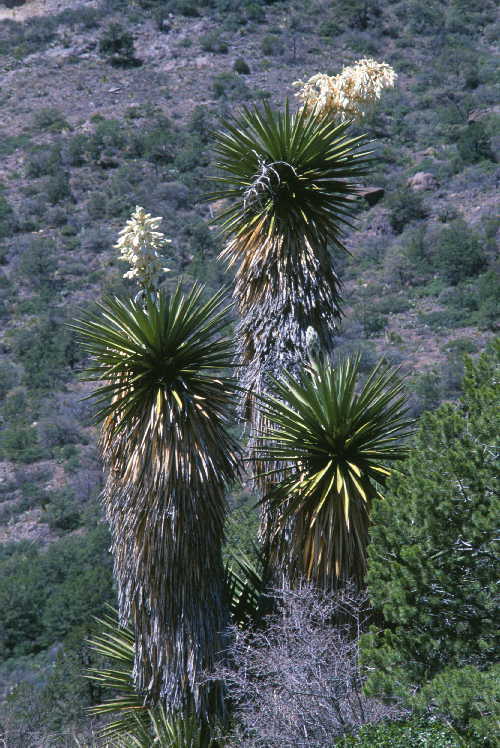In the image, three tall, spiky yucca plants dominate the foreground, each with distinctive features. The tallest yucca leans sharply to the right and showcases a spike adorned with small yellowish-white flowers. The second tallest stands upright, also in full blossom with similar white flowers, while the shortest one hints at budding flowers that have yet to bloom. The yuccas are characterized by their long, thin, and spiky leaves forming spherical clusters at the top, with their trunks displaying a coarse, thatch-like texture, colored in shades of gray and light brown. At the base of the yuccas, thorny, gray bushes devoid of foliage can be observed. To the right, a small coniferous tree with green foliage adds contrast to the scene. The background reveals a barren, light brown desert landscape dotted with green, short bushes. This daytime photograph captures the rugged beauty of these plants thriving in their natural habitat.